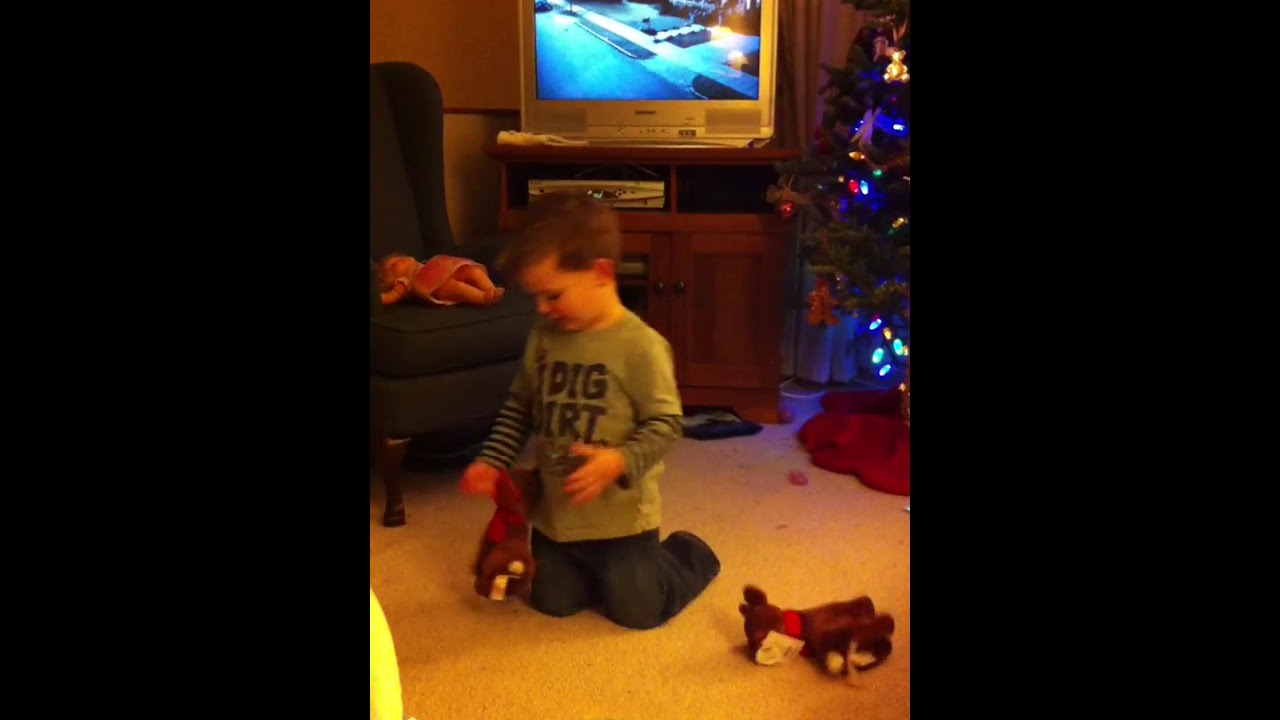In a cozy beige-carpeted living room adorned for Christmas, a little boy with short light brown hair kneels intently on the floor. Dressed in a grey t-shirt emblazoned with "Dig Dirt" and layered over a long-sleeve striped shirt, as well as blue jeans, he focuses on a brown plush reindeer toy with a red bow. Nearby, a second similar plush reindeer lies on the carpet. Behind him, a small, lit Christmas tree with blue lights and ornaments sparkles, standing next to a brown wooden entertainment stand. The stand, featuring drawers and shelves, holds a silver VCR underneath an old-fashioned silver CRT television that is turned on. To the left of the boy, a blue upholstered armchair cradles a baby doll, adding to the festive and homey ambiance of the room.